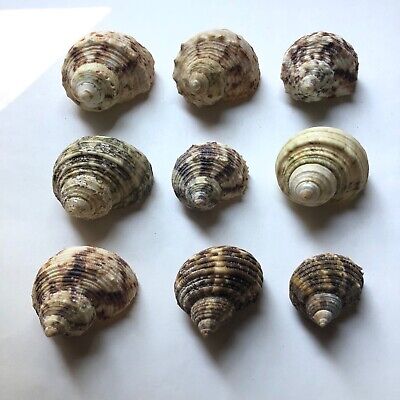The image features a precisely arranged collection of nine seashells displayed on a bright, sky-blue background, possibly a flat surface like a table or floor. The seashells are positioned in a perfect 3x3 grid, each pointing towards the viewer with their tops tapering to neat points. These shells, resembling conical cockles, showcase a calm gradient of colors including off-white, light brown, medium brown, dark brown, and various shades of green ranging from light to dark. Detailed ridges and bumps adorn the curves of these spirally shells, emphasizing their natural texture. All the shells are impeccably intact, uniformly sized, and exhibit a combination of earthy and subdued hues, creating a harmonious visual contrast against the bright blue background.